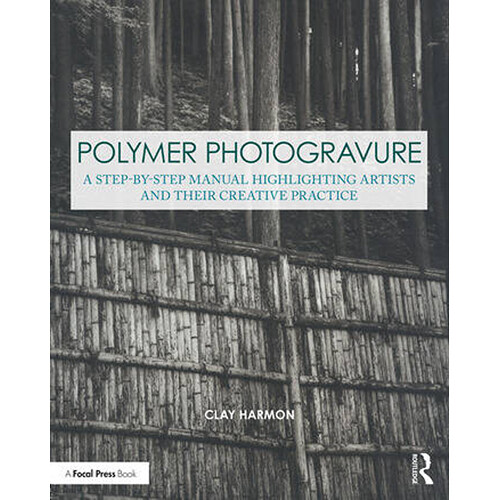The image depicts the black and white cover of a book titled "Polymer Photogravure: A Step-by-Step Manual Highlighting Artists and Their Creative Practice." The cover features a tall wooden fence, constructed from vertical bamboo-like poles and horizontal supports, in the foreground. Behind this fence, there is a dense forest with slender tree trunks and thick underbrush that obscures the sky, suggesting a deciduous backdrop on a hillside. Text on the cover includes the title "Polymer Photogravure" in green over a white background, followed by the subtitle in blue. At the bottom, the name "Clay Harmon" appears prominently in white text, surrounded by additional information: "a focal press book" in black text within a white box on the bottom left, and an unspecified imprint showing a person's head in profile on the bottom right.